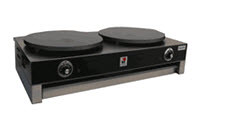The image depicts a product photograph featuring a DJ's turntable setup, prominently displayed against a stark white background, suggesting its use for online storefront listings. The turntables are positioned side by side on a sleek, black base adorned with various black knobs and controls. Despite the photograph's small, thumbnail size, it is clear that the background has been purposefully left blank to emphasize the product. A logo is visible on the equipment, although its details remain indistinguishable due to the image's minimal dimensions. The overall aesthetic of the turntables is highly polished and uniform in color, suggesting a professional-grade DJ setup designed for efficiency and style.